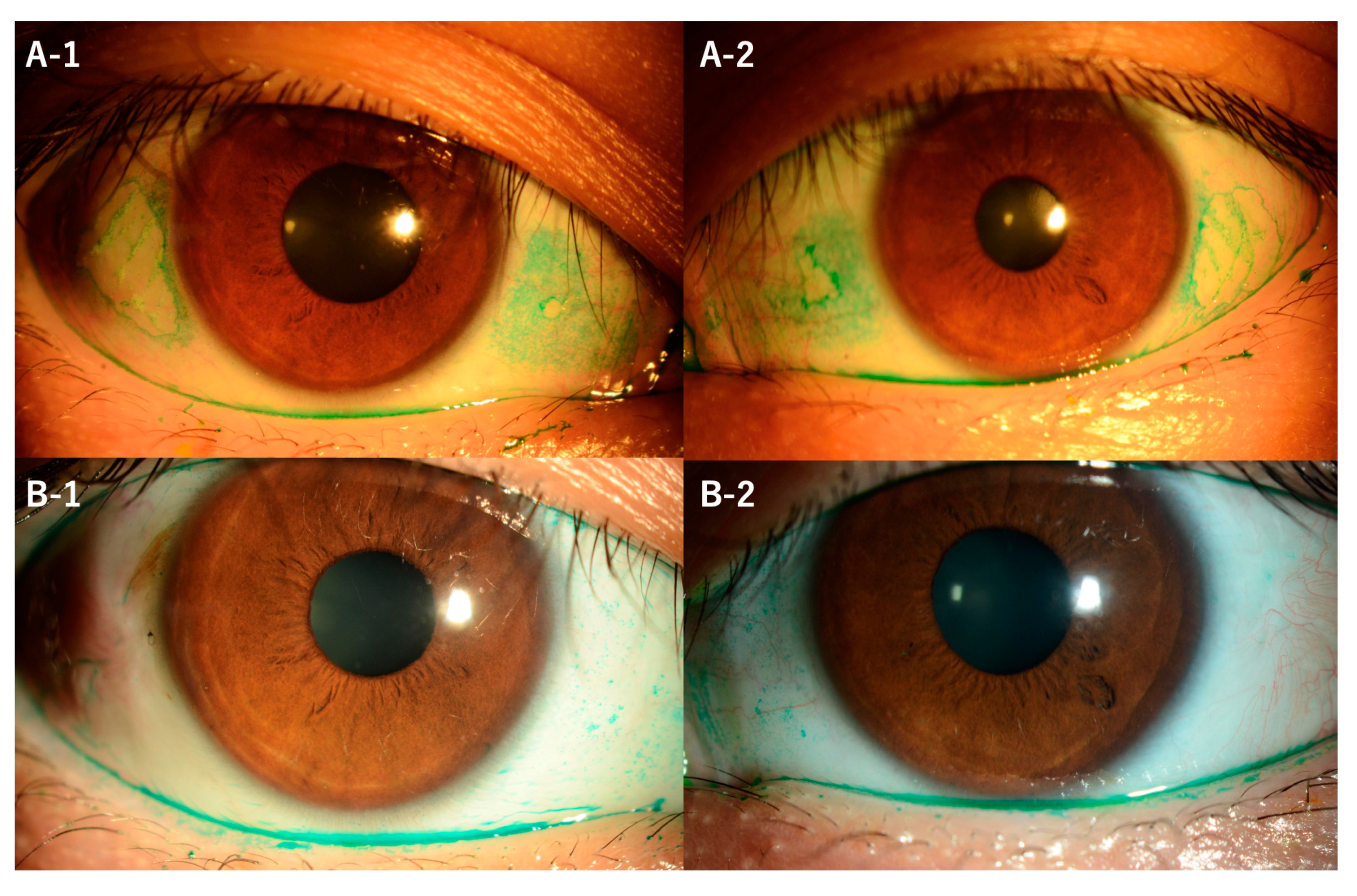The image is a large composite consisting of four smaller pictures of brown eyes, each labeled and positioned distinctly. The top row features images labeled A1 and A2. The bottom row includes images labeled B1 and B2. 

- In the top left (A1), there is a close-up of a brown eye with a noticeably dilated pupil. The sclera (white part of the eye) has patches of green/teal dye, and black eyelashes are clearly visible. The entire image has a subtle yellowish hue.
- The image in the top right (A2) shows a similarly colored brown eye with a smaller, less dilated pupil. Similar green/teal dye is present in the sclera, and the black eyelashes are still prominent. This image also retains the yellowish hue.
- The bottom left image (B1) features a lighter brown eye, attributable to differing lighting conditions. The pupil is smaller, and the amount of green/teal dye in the sclera is minimal. There is a red discoloration on one side of the eye, which is not as apparent in the other images.
- The bottom right image (B2) presents a brown eye with a slightly larger pupil compared to B1. The green/teal dye is mostly faded, visible only in minimal amounts. There are signs of redness, particularly on both sides of the eye, with a purplish tint on the left side.

The overall image sequence seems to document variations in pupil dilation and the distribution of dye within the sclera under different lighting conditions.